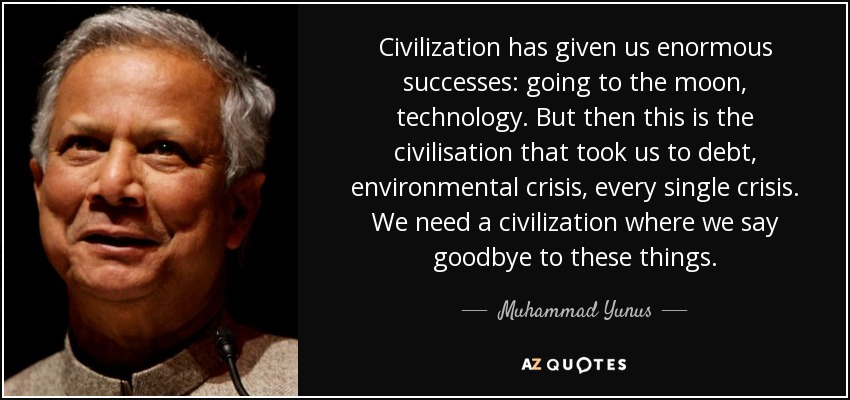The image depicts an old man, Muhammad Yunus, the founder of micro lending, against a black background. On the left side of the rectangular image, his face is prominently featured. He has gray, short hair and is smiling lightly. He wears a beige suit with a high collar, and you can see up to the tips of his shoulders. Positioned in front of a microphone, he looks like he’s about to deliver a lecture.

On the right side of the image, a paragraph in white font contrasts sharply with the dark background. The quote reads: "Civilization has given us enormous success: going to the moon, technology. But then this is the civilization that took us to debt, environmental crisis, every single crisis. We need a civilization where we say goodbye to these things." Underneath, his name, Muhammad Yunus, is handwritten in cursive. Below the paragraph, the logo "AZ Quotes" appears, with the "Z" in yellow and the rest of the letters in white, adding a touch of color to the otherwise monochromatic scheme. The overall tone of the image conveys a sense of depth and seriousness.